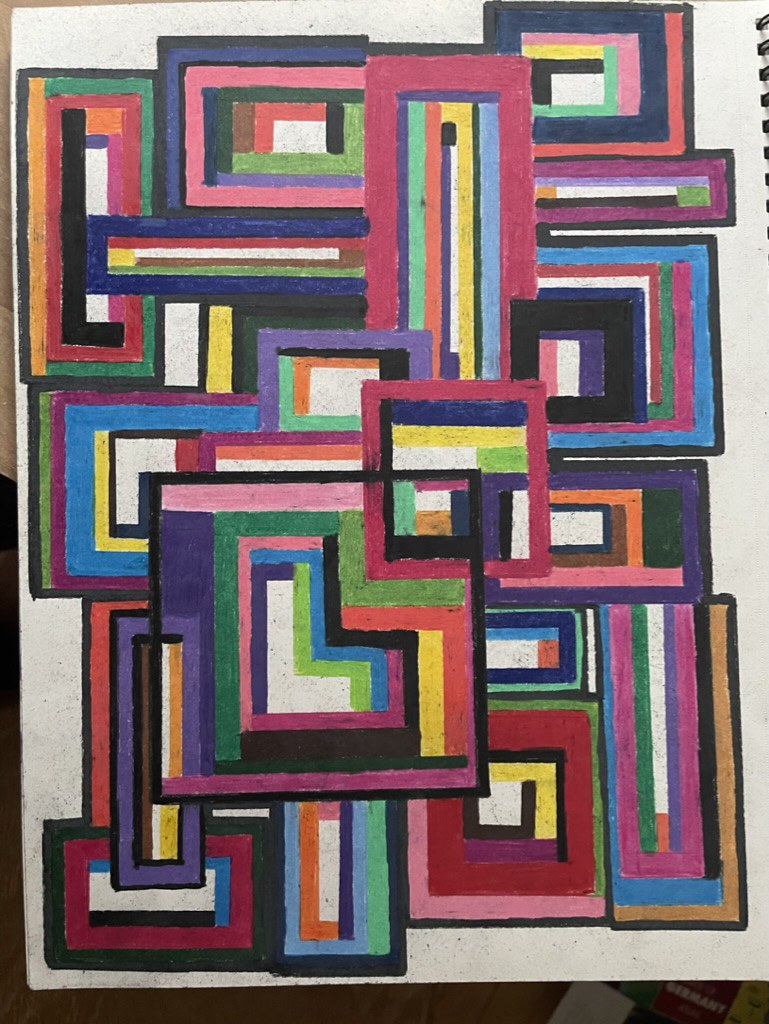This image showcases a vibrant, abstract work of modern art, possibly created with crayons or pastels. The composition is a striking array of geometric shapes, primarily rectangles and squares with sharp edges, covering approximately 90% of a white canvas or paper. These shapes are filled with a plethora of colors from the entire spectrum, including orange, yellow, pink, green, blue, purple, red, and black, and are mostly outlined in black. The shapes overlap in a multi-layered arrangement, densely populating the central area. A notable feature is an L shape formed by these colorful blocks, with no discernible pattern. Slight portions of the white background remain visible, along with a distinct brown patch on the bottom left and three small objects—red, yellow, and white—in the bottom right corner, presumably resting on a floor. Additionally, in the upper right corner of the photo, black rings holding the paper to a notebook are visible, adding a touch of structure to the composition.